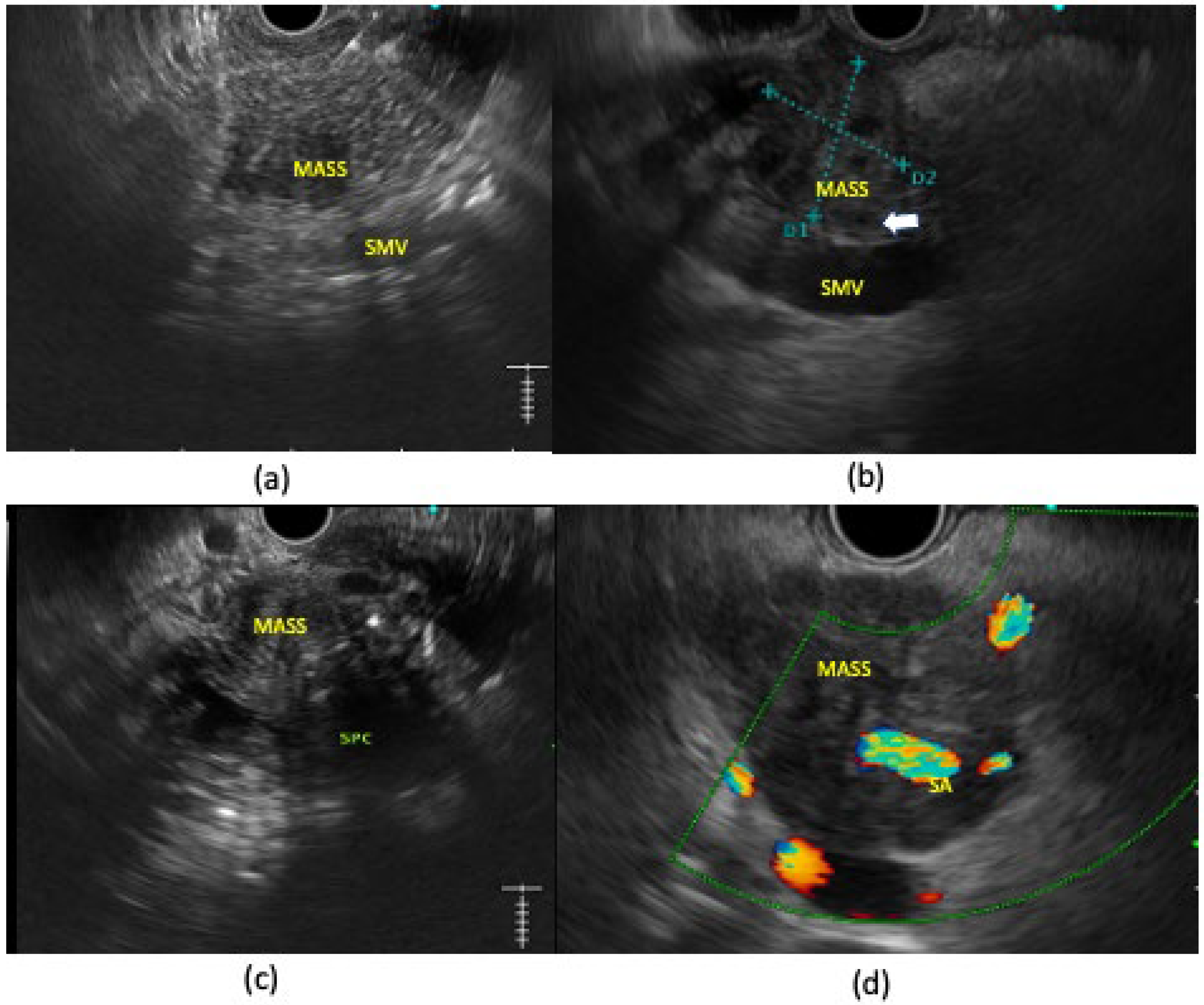The image contains four black-and-white ultrasound scans, each labeled respectively with a small black letter: A, B, C, and D. These scans are arranged in a 2x2 grid with A and B on the top row and C and D on the bottom row. Each scan features a radial pattern with a central black circle, surrounded by concentric gray and white patches.

In image A, yellow text labels denote "mass" and "SMV," with SMV appearing to the left and somewhat below "mass." There is a vertical measuring line on the bottom left, intersected by smaller horizontal lines, and capped by a long horizontal line on top. 

Image B similarly labels "mass" and "SMV," this time with SMV directly beneath "mass." Blue dotted lines, labeled D1 and D2, crisscross each other, and a white arrow points to an area between "mass" and "SMV."

In image C, the label "mass" is again present in yellow, while "SPC" appears in green to the left and below "mass."

Finally, image D also contains the "mass" label, with the addition of various multicolored patches including green, orange, yellow, and red. The green outline demarcates an area with a radial shape that has a flat left side. 

The combination of text labels, color coding, and measuring lines across the scans suggest a detailed examination and identification of specific anatomical features or anomalies.